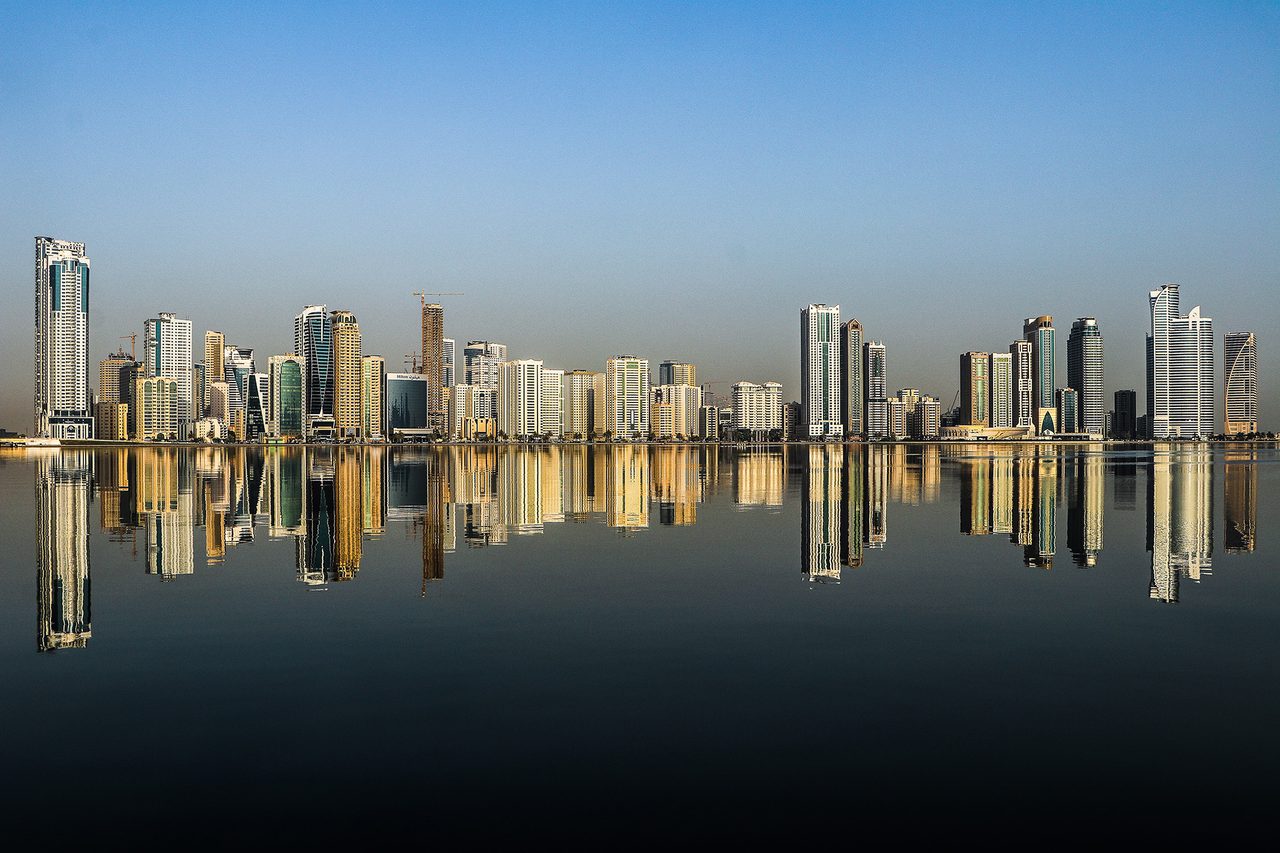This detailed photograph captures a serene and pristine cityscape during the daytime. The focus is a coastal city with numerous high-rise buildings of varying heights, shapes, and colors—predominantly white, with hints of dark brown and blue—giving the skyline a dynamic appearance. The tall, concrete buildings stretch horizontally across the center of the image, creating a clear division between the top and bottom halves. Just below the buildings, there appears to be a strip with some small trees, likely indicating the presence of a road. The sky, taking up the top half of the photograph, is a stunning clear blue, subtly gradient to gray near the horizon, and is completely free of clouds. The bottom half showcases a perfectly still ocean, mirroring the entire cityscape with almost no distortion, creating an almost exact reflection of the city and reinforcing the calmness of the scene. The absence of boats, ripples in the water, birds, or any disturbances makes the reflection in the water strikingly clear, suggesting either a rare moment of tranquility or potential graphical manipulation. This horizontal rectangular photo artfully balances the elements of sky, city, and water into a cohesive and visually compelling image.